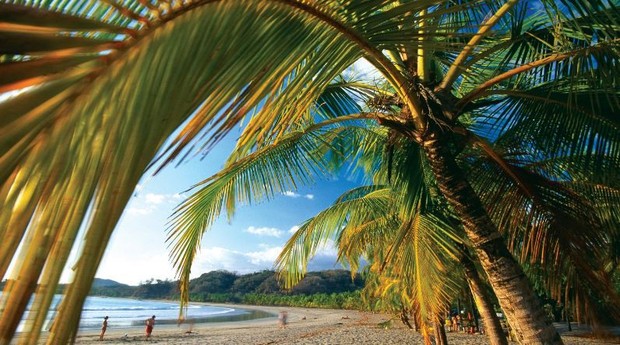This vibrant color photograph captures a picturesque tropical beach scene. The foreground prominently features a large palm tree with a dark, curving trunk and lush fronds extending towards the camera, creating a natural canopy that frames the vista. The palm fronds vary in color from deep green to golden brown, adding rich texture and dimension. Beyond the tree, the scene opens up to a wide sandy beach with a beige hue, lightly dotted with footprints. The ocean's gentle waves lap at the shore, a serene lagoon of light blue water.

In the distance, verdant hills covered in dense green vegetation form a beautiful backdrop, meeting a sky that transitions from a lighter blue on the left to a darker shade on the right, punctuated by puffy white clouds. Amidst this tranquil setting, three people are visible on the beach, a man and a woman walking along the shore and another small group off to the right, under a grove of trees or possibly near a surfboard shop. Some suggest additional figures can be seen under a gazebo or among the trees, but they remain indistinct.

The photograph was likely taken in a tropical location, possibly Hawaii or a remote Latin American beach, exuding an inviting, happy atmosphere perfect for a vacation. The palm trees' proximity and the vivid details of their fronds make the viewer feel as if they could almost reach out and touch them, adding an immersive quality to the image.